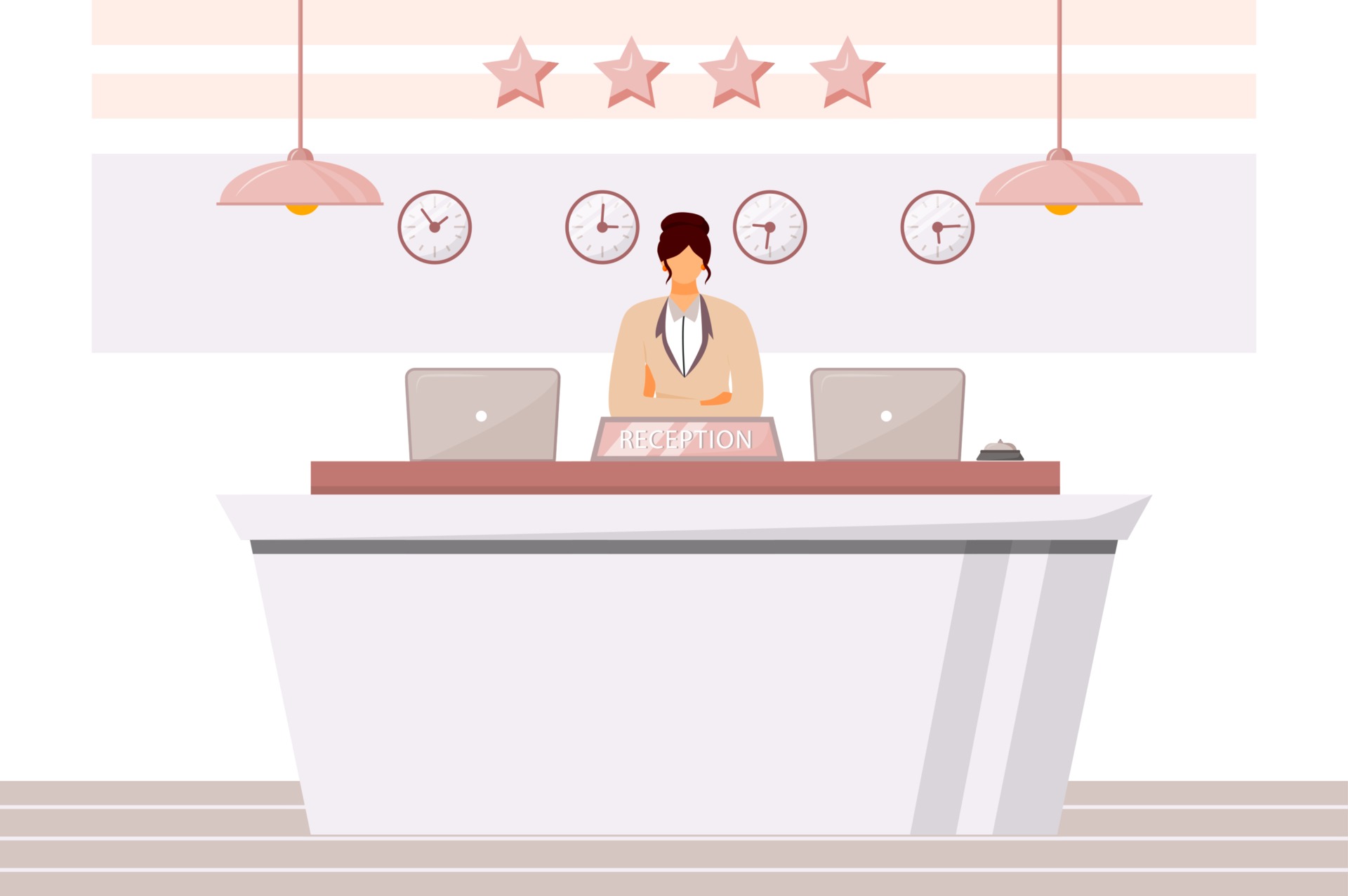The image is a minimalist, digital illustration of a reception area, likely designed for online use such as in a video or graphic presentation. At the center is a female receptionist depicted with brown hair tied in a bun and tendrils extending from it. She is dressed in a peach suit coat over a white collared, button-up shirt, and her facial features are notably absent, resulting in a simple, peach-colored face. Her arms are crossed and rest on a gray desk marked with the word "Reception."

The scene is composed with a symmetrical balance: two computer monitors flank the receptionist on both sides of the desk, which also features a small gray bell. Suspended above are two dome-shaped, pink lights. Behind the receptionist, four clocks hang on the wall, each displaying a different time, adding an element of intrigue. Above the clocks, there are four stars. The color palette of the image is restrained, focusing on shades of gray, light reds, and variations of peach and salmon. The design elements are kept minimalistic, with simple rectangular patterns on the floor and back wall, enhancing the overall clean and uncluttered aesthetic of the illustration.